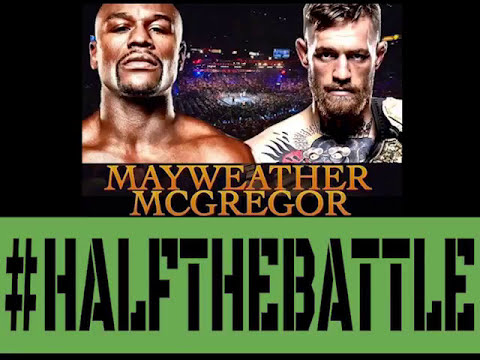The image is a fight announcement poster featuring Floyd Mayweather and Conor McGregor from the neck up in a face-off pose. Floyd Mayweather, on the left, is a black man with a stern expression, sporting a thin goatee and no visible tattoos. On the right, Conor McGregor, a white man with a swooping fringe, has prominent ears, facial hair including a mustache and short beard, and tattoos covering his chest. The fighters are positioned against a background that shows a distant view of a crowded fight stadium, highlighting a boxing ring in the center. At the top, in orange serif text, "Mayweather" and "McGregor" are displayed in two lines. The bottom third of the image features a green rectangle with black capitalized text reading "#HALFTHEBATTLE," all combined into one word. The overall palette includes black borders surrounding the main visual.